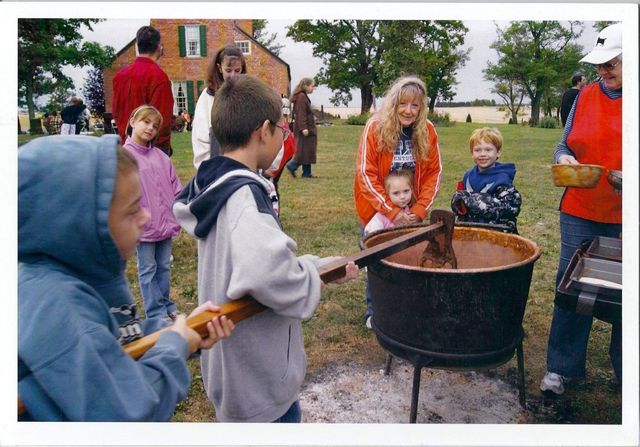This horizontally aligned rectangular picture, bordered thinly in gray on three sides with a black border on the right, captures a vibrant family gathering outdoors on a grassy area with hints of yellow patches and concrete pavement. Central to the image is a large, black, circular kettle perched on a black metal stand with three or four legs. Its interior appears charred with remnants of a fire, ash, and some red-brown substance, possibly chili. Two children in the foreground, dressed in blue and purple hoodies and blue jeans, are engrossed in dipping a long wooden rod with a metal end into the kettle.

To the left, a woman with long blonde hair, clad in an orange and white shirt over a blue top with white text, holds a small girl dressed in pink; a red-haired child in a blue hoodie and a camouflage-patterned coat stands next to her. Behind the pot, to the right, a man in a distinct orange vest over a blue and white striped shirt, blue jeans, and a white hat, observes the scene while holding a pan.

In the background, a mix of adults and children adds to the lively atmosphere. Among them, a man in red and a woman in a brown coat and blue jeans are noticeable. Overlooking this assembly is a large, two-story brown brick house with white windows and green shutters, set against a sky mixed with white and blue hues. The yard is scattered with green trees, adding a comforting natural backdrop to this scene of familial bonding and culinary activity.